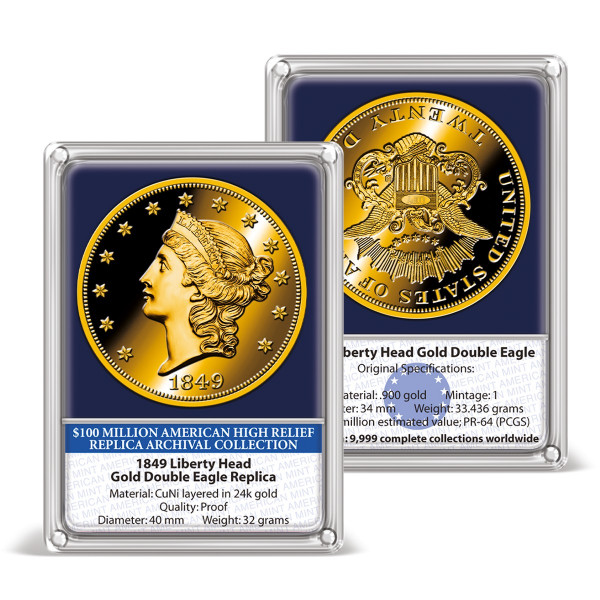This product photograph showcases a meticulously detailed replica of the 1849 Liberty Head Gold Double Eagle coin, encapsulated in a clear rectangular acrylic case. The coin's front and back are presented side-by-side against a solid white background, creating the illusion of floating in an empty, featureless void—a common technique in commercial presentations for online shops, listings, websites, or catalogs. The coin is prominently displayed against a piece of blue round fabric with cutouts, ensuring visibility of both sides.

The obverse side of the coin, shown on the left, features a detailed engraving of Lady Liberty's profile, characterized by long wavy hair and a tiara. Surrounding the portrait are a series of star engravings, with the date "1849" etched at the bottom. The coin's rich, golden-yellow hue is vividly captured against the contrasting blue fabric.

The reverse side, displayed on the right, showcases an engraving of an eagle with extended wings, encircled by the words "United States of America." Notably, this side of the coin appears upside down within the display. A small tag beneath both images identifies the coin as part of the "$100 million American High Relief Replica Archival Collection."

Additional descriptive tags provide further details: the front label describes it as a "1849 Liberty Head Gold Double Eagle replica," made from copper-nickel layered in 24-karat gold, with the quality noted as 'proof.' The diameter of the coin is listed as 40 millimeters, with a weight of 32 grams. The back description references the original specifications, including the material as 90% gold, and an estimated value that underscores the coin's historical and collectible significance.